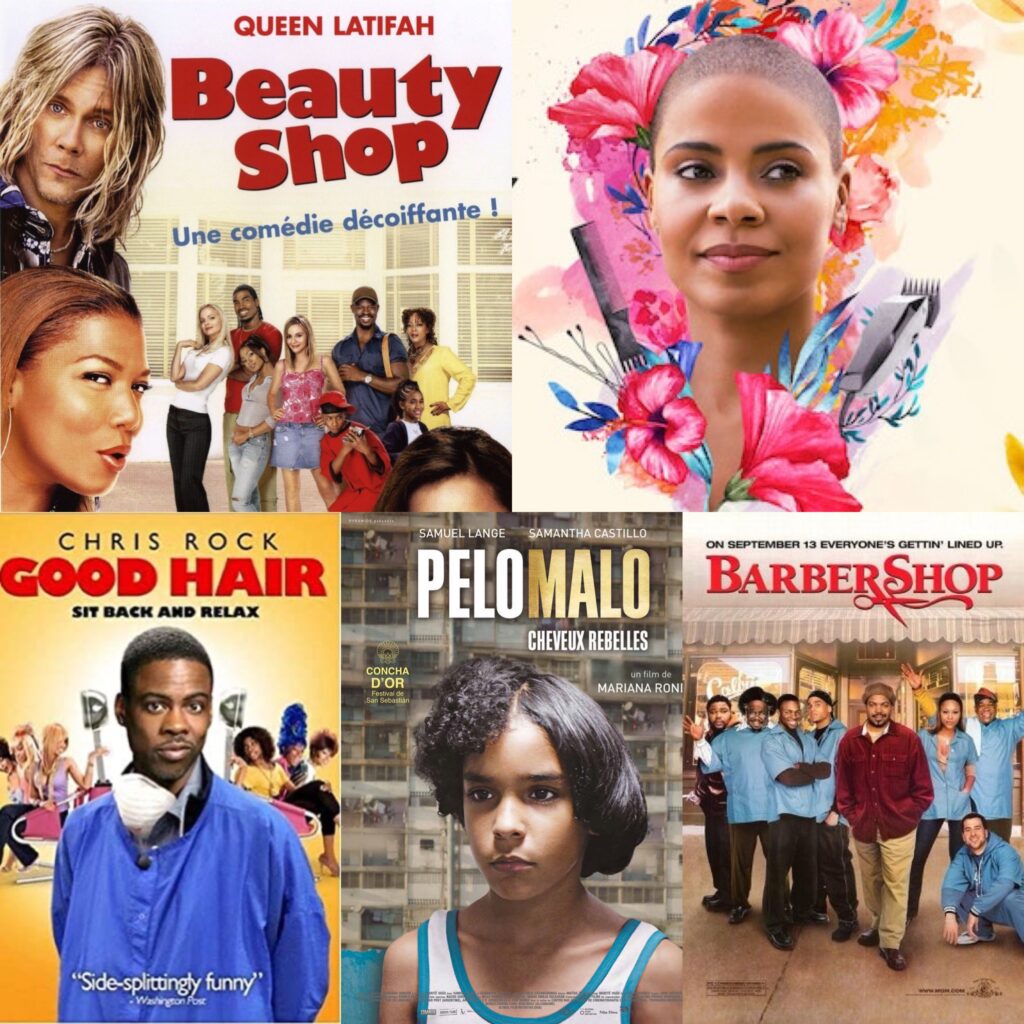This image is a composite poster, assembling five different movie covers in a photo grid. In the top left corner, there is a poster with bold red text that reads "Queen Latifah: Beauty Shop," accented by the French phrase "Un Comédie Décoiffante." This section features several people against shutters with Queen Latifah making a funny face and a man with long blondish-brown hair looking straight at the camera.

To the right is an image of a dark-complected woman with a shaved head, surrounded by vibrant flowers in pink and blue hues against a yellow background. Close to her right is a comb, while hair clippers are on her left. She has dark eyelashes and is looking to her side, maintaining a calm demeanor.

Below these two posters, three additional movie covers are lined up. On the left is "Chris Rock: Good Hair," highlighted by the phrase "Sit back and relax" and "Sidesplittingly funny." Chris Rock is depicted wearing a blue smock and a white towel around his neck, with hairdryers and people in the background.

The middle cover showcases a movie titled "Hello Mellow Curlux Rebels" featuring a black woman in a blue and white tank top. Her hair is styled asymmetrically, with straight hair on her left side and curly hair on her right, set against what appears to be apartment buildings.

Lastly, to the right is a poster for "Barbershop," which reads, "On September 13th, Everyone's Getting Lined Up." This image displays seven men in blue shirts and dark trousers, standing behind Ice Cube, who wears a red flannel shirt and khaki pants. Ice Cube appears to be the prominent figure, indicative of his leading role in the film.